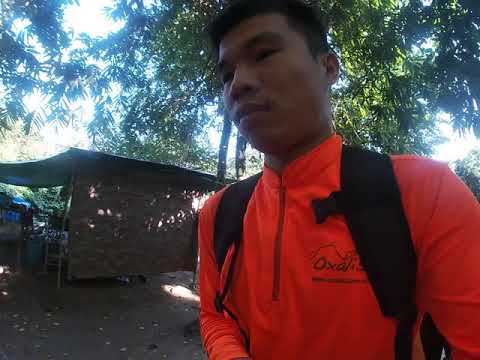In this selfie, an Asian man with short black hair is seen walking through a lush, forested area during the daytime. Sunlight filters through a dense canopy of green leaves overhead, casting a bright yet shaded light on the scene. The man is in the foreground, wearing a vibrant orange zip-up long-sleeve shirt with black lettering on the shoulder, partially spelling "OXCALIS." He also sports a black backpack with unbuckled straps. Behind him, to the left side of the image, there is a tented area with a piece of plywood serving as a wall, and various tables and carts laden with snacks and refreshments, suggestive of a makeshift market stall or campsite. The area has a tropical ambience, with diverse trees and lush vegetation forming a natural backdrop.